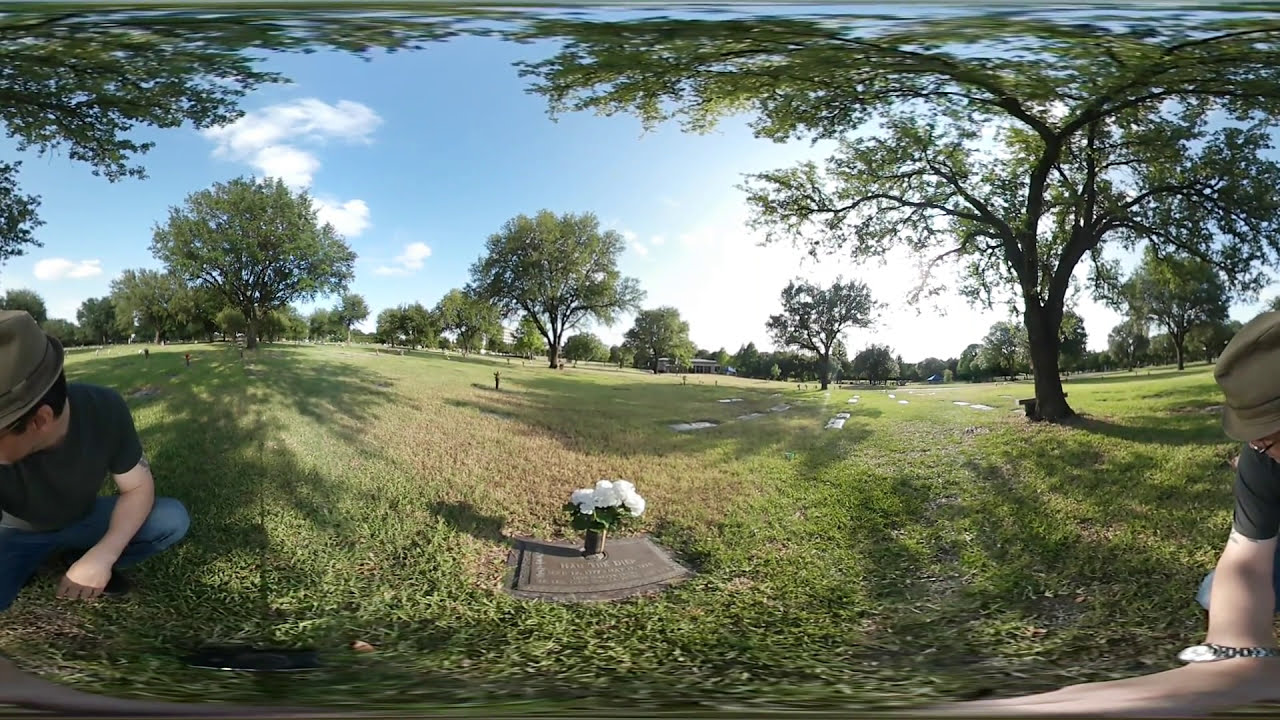The photograph appears to be taken in a serene cemetery on a sunny day with blue skies and a few white clouds. The image prominently features a middle-aged man, approximately in his early 30s, wearing a green fedora with a tan leather headband, glasses, a black t-shirt that partially reveals a tattoo on his right bicep, and blue denim Levi jeans. He is captured squatting down, focused intently on a flat grave marker adorned with a white vase filled with fresh white flowers. The picture has a panoramic effect, making it appear as though the left side of the man connects with the right side, emphasizing his presence on both sides of the image. Surrounding him are lush green grassy areas with patches of dead grass near the gravestone, and a scattering of green leafy trees that provide shade over the man and add to the peaceful atmosphere. In the distance, other flat graves and a low-lying building can be seen, but he appears to be the only person present, tenderly attending to the gravesite. The overall scene is both reflective and somewhat distorted, due to the unusual panoramic effect, lending a unique, almost surreal quality to the photograph.